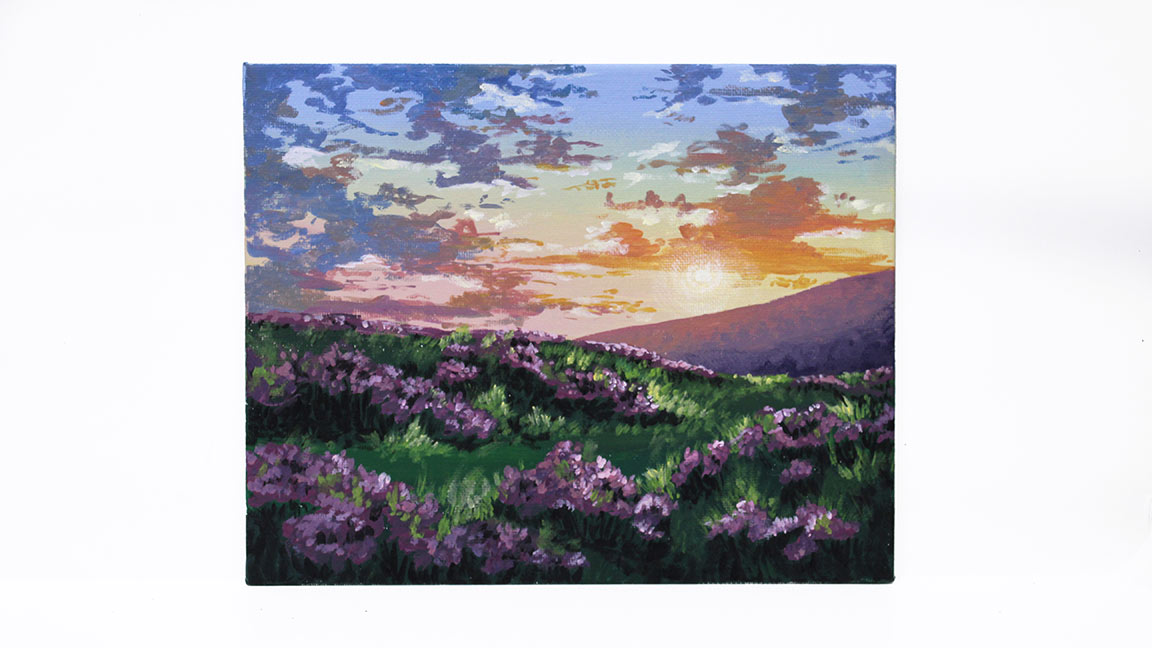This painting by Anand Sherit depicts a serene landscape of an open field on gently rolling slopes. The field is primarily green grass interspersed with clusters of vibrant purple flowers, which dominate the foreground. The sky, taking up the upper half of the painting, portrays a beautiful transition of colors as the sun sets, casting warm hues of orange, yellow, and a hint of purple onto the clouds. The sun is partially hidden behind an orange cloud near the right side of the image, illuminating the sky with a dimming, yellowish glow. In the background, a distant, dark purple hill stretches from the right towards the center, anchoring the sunset scene and providing depth to the composition. The interplay of vibrant floral fields and the warm, fading sunlight creates a tranquil and captivating mood.